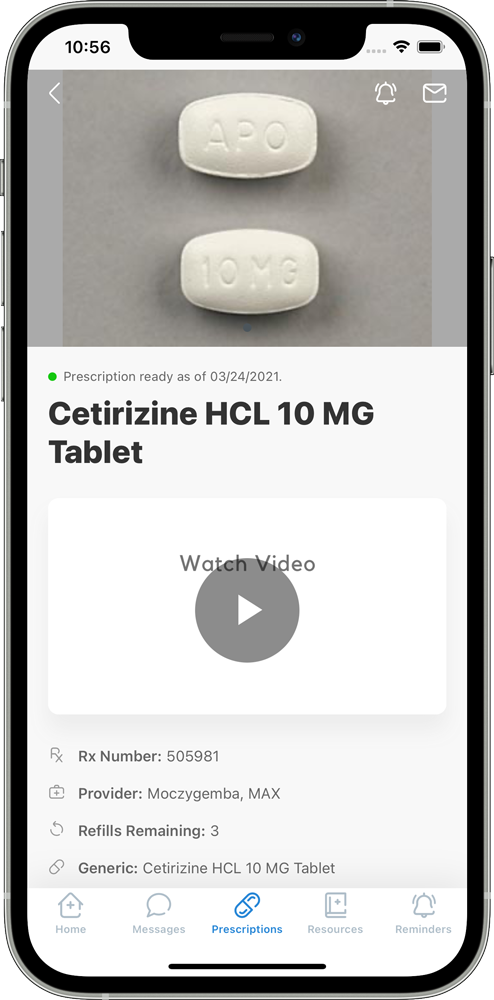This is a detailed screenshot of a smartphone displaying a digitally manipulated interface. The smartphone has distinct black bezels with slightly transparent edges, suggesting it is encased in a protective cover. On the left side of the device, there are three buttons, while an unusual solitary button is located on the right side. At the top of the screen, there is a small lens intended for taking selfies.

The interface shows a typical smartphone status bar: the upper-left corner displays the time as 10:56, while the upper-right corner indicates both a full battery and a strong Wi-Fi connection, set against a white background.

Immediately below the status bar is a photograph of two white, oval-shaped pills on a gray surface. The top pill is inscribed with "APO," and the bottom pill is marked "10MG." In the upper-left corner of the photo, there is a white left-facing arrow. The upper-right corner contains two icons: a bell for notifications and an envelope to represent email.

Beneath this image, the interface features a white area with text, which reads "Prescription ready as of 03/24/2021."